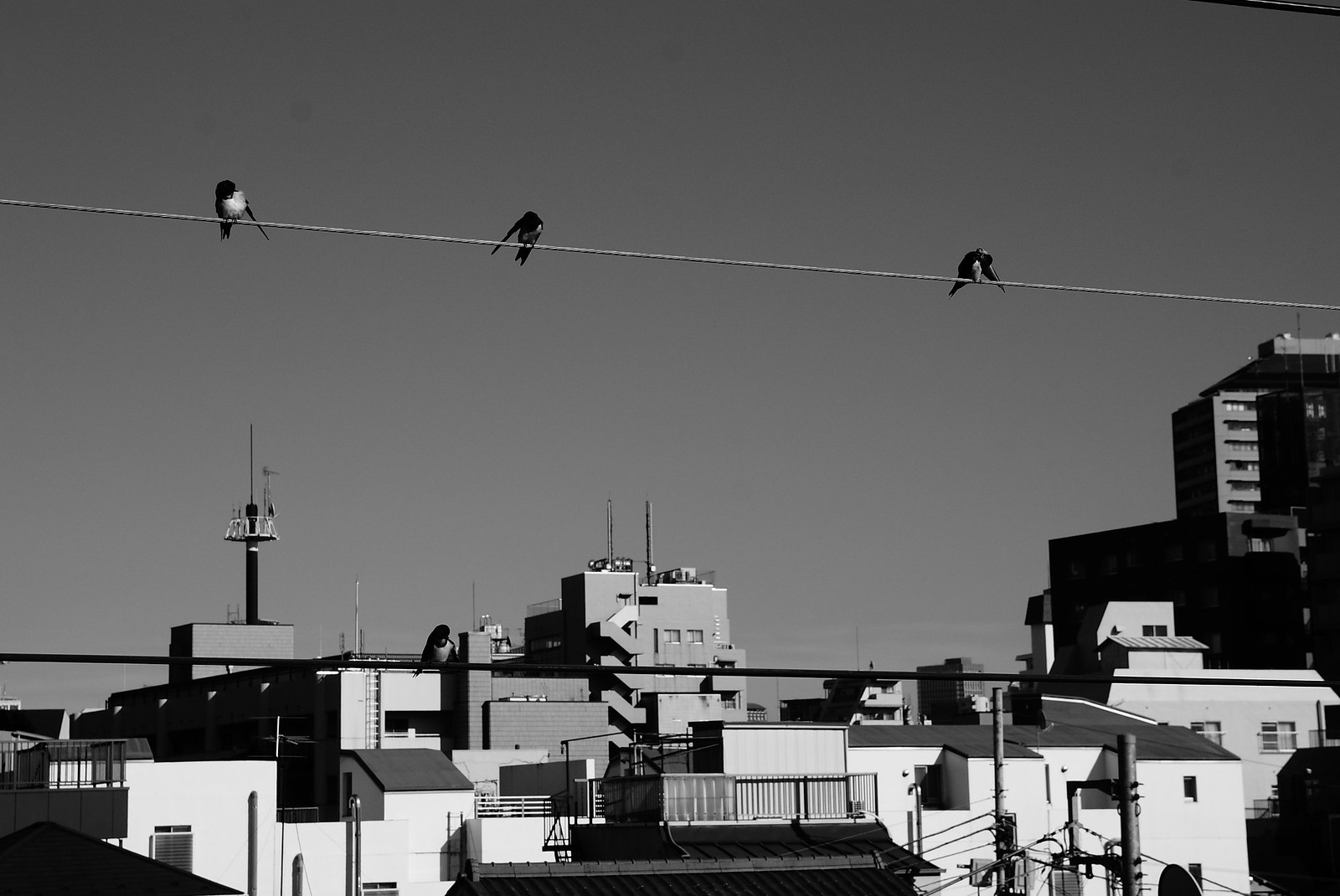A black and white photograph captures a cityscape under a clear, sunny sky. The upper two-thirds of the image is dominated by a gray sky, interrupted by a power line stretching horizontally from right to left, hosting three perched birds. These birds exhibit intriguing postures: the leftmost bird, with a dark head and white breast, faces the camera, while the middle bird faces away. A significant gap separates these two from the bird positioned just right of center. To the left of the composition, there's a pole supporting the power line, accompanied below by various buildings. Closest to the left, a small white building stands near a large, gray edifice with a tower in its back left corner. Adjacent to these, a narrow, taller building with a small tower tops the skyline, followed by a longer white building with a dark slanted roof. Nearly off the right edge, another white structure with distinctive windows is visible, crowned by a small rooftop structure, and shadowed by a towering building behind it, which extends past halfway up the photograph. Highlights from the sunlight illuminate the sides of these structures, adding depth and life to the cityscape.